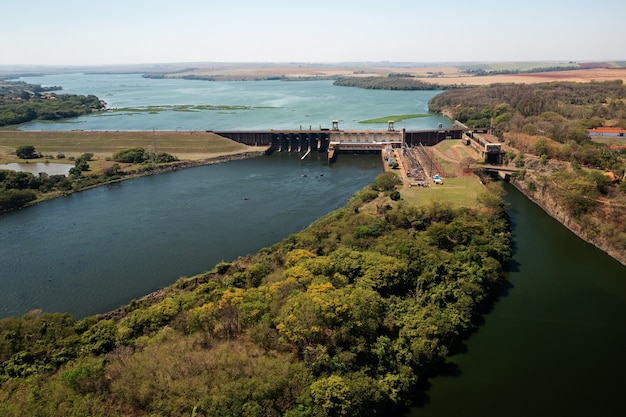The image is an expansive aerial view, likely captured by a drone, illustrating a large hydroelectric dam and its surrounding landscape. Dominating the scene, the dam appears solid and concrete, extending across a wide stretch and creating a substantial reservoir of light blue water. This reservoir, situated higher at the back of the image, contrasts starkly with the darker shade of water in the lower foreground, divided by the impressive structure of the dam.

The dam itself separates two distinct bodies of water, with what appears to be an island-like landmass in the middle. This central stretch of land features multiple small buildings, likely houses, alongside a sizeable parking lot. Nearby, a notable building structure, white with orange accents, stands out on the right side of the image.

Flanking the water bodies, the landscape is varied, with green fields, trees, and bushes spread throughout. The terrain is mostly flat and beige, indicating large expanses of fields. Underneath the camera, a wooded area adds further greenery to the composition. The vast blue sky forms a serene backdrop for this intricate interplay of manmade and natural elements.